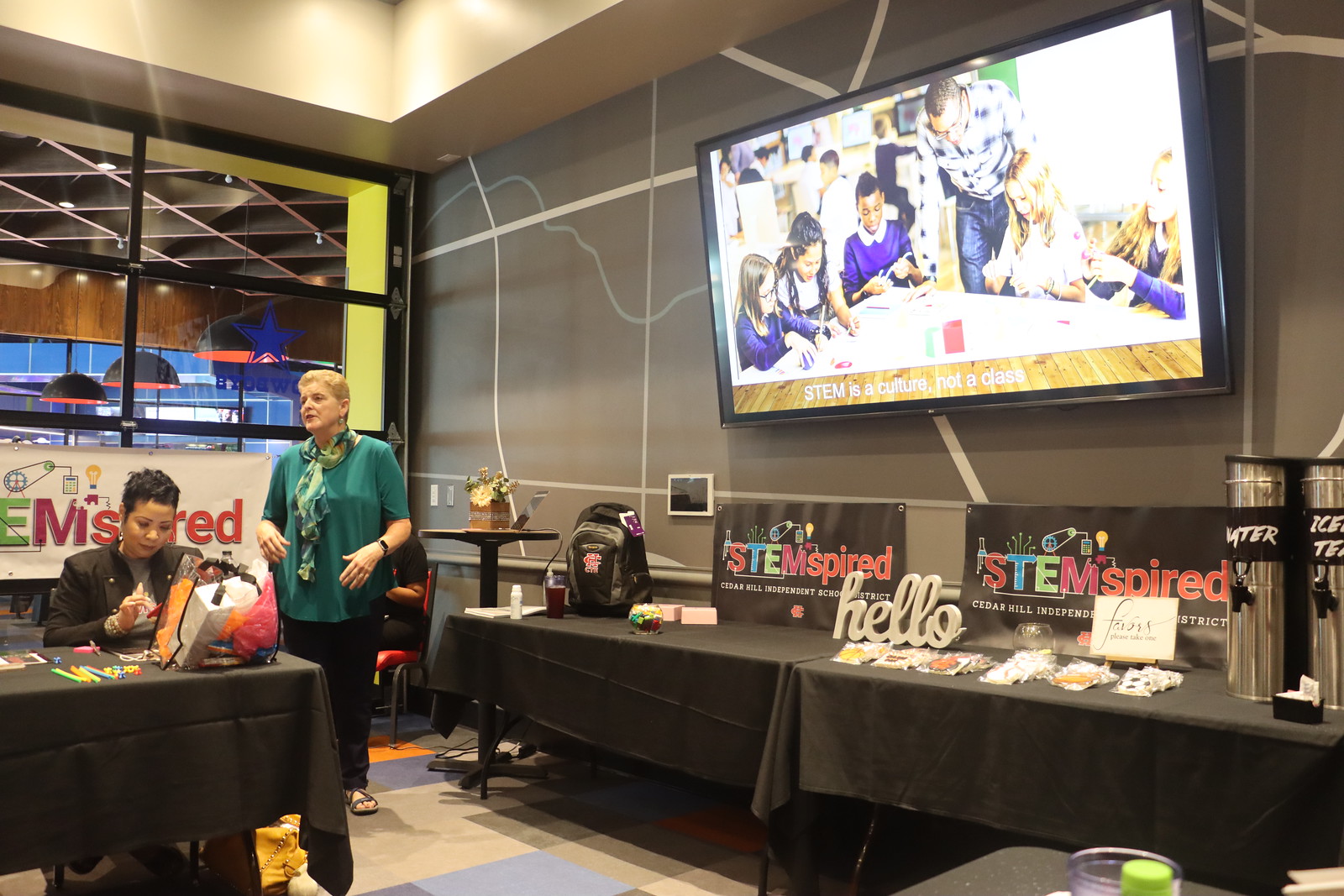In a spacious college hall brimming with natural light from the large windows, a notable event or convention appears to be taking place. At the center of activity, an older woman in a green shirt and black pants stands behind a slightly younger woman in a black blazer, who is seated and focused on some work at one of the several tables draped in black cloths. These tables are adorned with a mix of snacks, iced tea dispensers, coffee pots, and signs in colorful letters reading "STEM Inspired." Scattered around are various items including backpacks, bags, and cups, indicating an engaged audience.

Behind them, a large flat-screen TV mounted on a gray wall displays the phrase "STEM is a culture, not a class," along with an image of an instructor guiding several children at a table, reinforcing the educational theme of the setting. The vibrant, communal atmosphere suggests a lecture or demonstration aimed at empowering women to join the STEM field, as evidenced by the attentive crowd and the collaborative efforts being showcased.